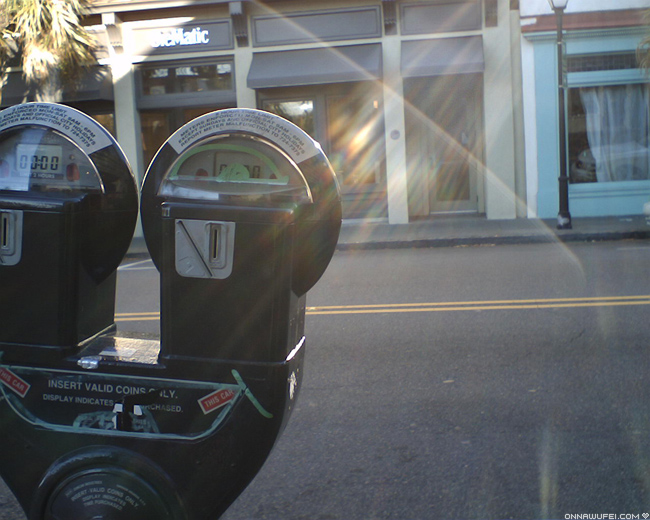The photograph, taken on a bright sunny day, captures an up-close view of a black parking meter standing on the sidewalk with two meters on top. The nearest meter is partly off-camera to the left, and the bottom extends off the bottom edge of the picture. The left meter shows partial visibility from the left side, while the right meter is fully visible. The parking meter includes a coin slot and a time display window; one of the meters shows remaining time while the other does not. A sticker on the machine reads "Insert valid coins only."

In the background, a well-lit street features two yellow center lines and is flanked by a sidewalk on the opposite side. Behind the parking meter, there's a black light pole a short distance from the right edge of the frame. Beyond the pole, a blue building with white-curtained windows stands next to a gray building with a dark gray awning, slightly obscured by bright sunlight. Modern storefronts populate the scene, with one identifiable by a white illuminated sign displaying partly visible text ending in "matic." This storefront is adorned with a teal hue and a door on the far right of the image. The overall setting is enhanced by reflected sun rays and occasional lens flares, adding a warm, hazy glow to the urban environment.